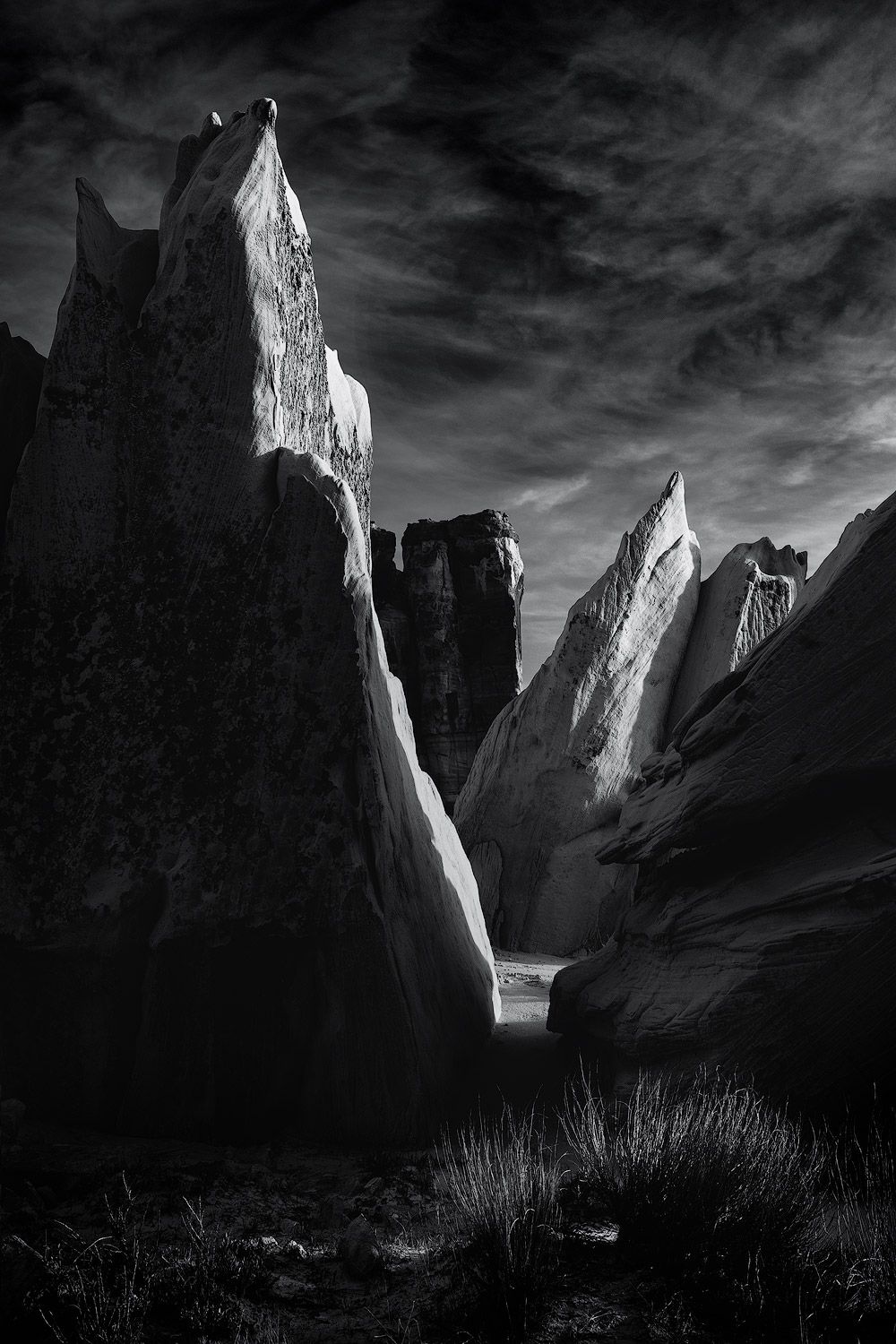This black and white photograph captures a dramatic landscape of tall, vertical rocky cliffs set against a heavily clouded sky. The towering rock formations, some of them spiky and formidable, rise steeply with little room at their peaks. The image, rich in shadow and shading, conveys a sense of rugged, unapproachable terrain, likely difficult to scale. In the lower right foreground, sparse prairie grass or small shrubs protrude, adding a touch of texture to the landscape. Though the scene hints at some illumination, particularly near the tops of the rocks where the light manages to pierce through, the overall atmosphere remains dark and somber. The sky is dominated by rolling, dark clouds, further enhancing the dramatic and desolate feel of this outdoor setting. There's no presence of people or animals, emphasizing the solitude and stark beauty of this natural environment.